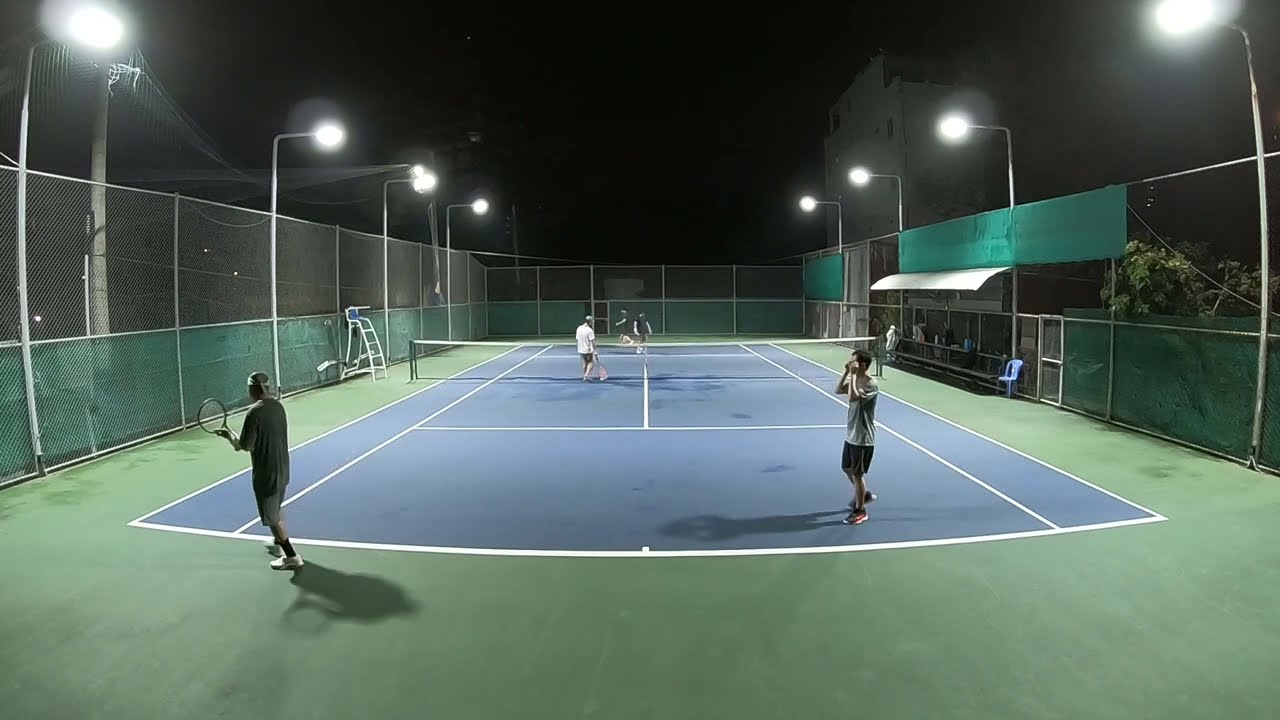In this nighttime photograph of an outdoor tennis court, the scene is illuminated by bright lights mounted on tall poles curving inwards, casting clarity on the vibrant colors and action below. The sky is pitch black, enhancing the stark contrast against the well-lit court. The tennis court itself features a blue playing surface with a green border, enclosed by a tall fence—its base lined with green padding. At the center of the court stands a net, partitioning the space where two sets of three players each are engaging in a game. They are dressed in a mix of casual workout clothes—some in gray, white, and dark shirts paired with black shorts. 

In the foreground, a player gripping a racket is notably visible. To the left of the net is a prominent white ladder chair for a referee. The right side of the court features benches sheltered under an awning, while beyond the fence, trees and a two-story gray building are faintly discernible. The overall ambiance suggests a lively evening match amidst a backdrop of dark sky and well-maintained facilities, encapsulating the essence of night tennis.